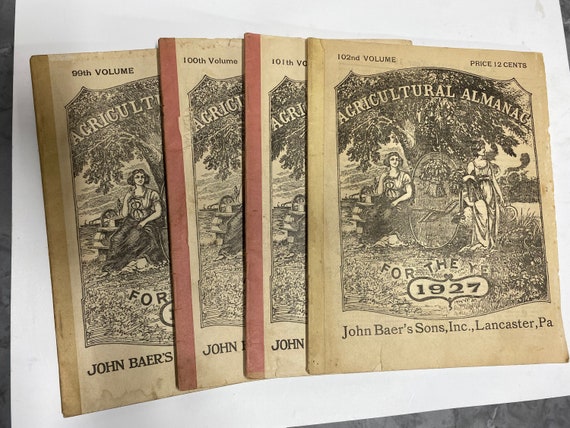The image is a color photograph depicting four vintage magazines laid out on a white sheet. These magazines, specifically titled "Agricultural Almanac for the Year 1927," were published by John Bayer's Sons Incorporated in Lancaster, Pennsylvania, and are nearly a century old, priced at 12 cents each. The volumes range from the 99th to the 102nd, indicated clearly on the upper left corners of each cover, albeit with a minor typo on the 101st volume, listed as "101th." The magazines are arranged in an overlapping fashion from right to left, with the top one on the right overlapping its neighbor, and so forth. The middle two magazines have orange bindings, while the outer two have a light brown, yellowish hue. Each cover features an identical, elaborate black-and-white illustration of a large tree with two women—one sitting under the tree and one standing on the other side. This illustration serves as an allegory for agriculture, further emphasized by the farm field in the background. The paper appears old and faded, adding to the photograph's vintage aesthetic.